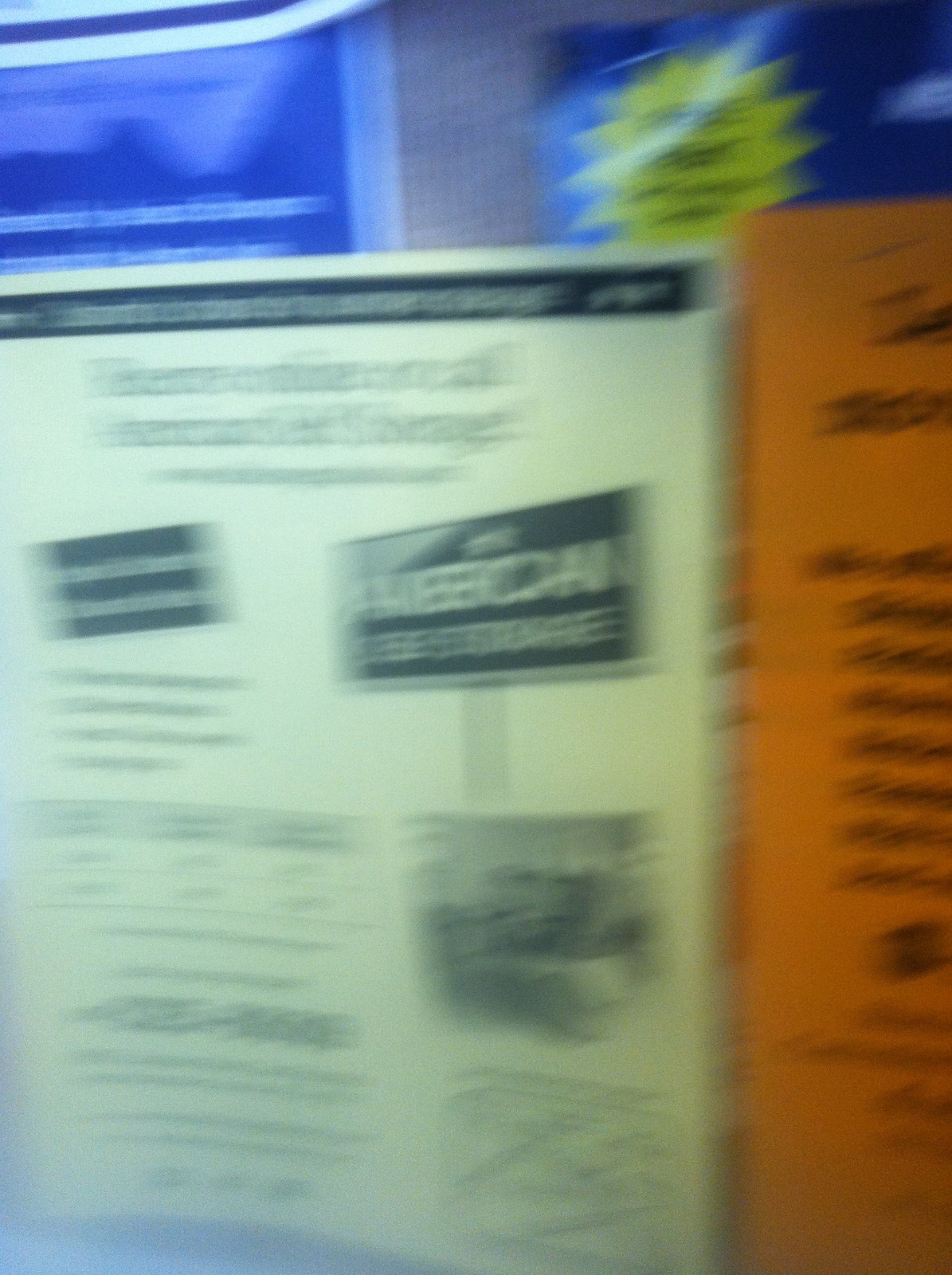A highly unfocused image captures several indistinct items. At the forefront, an off-white page features black text and a partially visible sign, possibly indicating "American" among other illegible words. Adjacent to this page is an orange sheet with unreadable black writing. The background reveals another nebulous object with a light blue section in the upper left corner. On the right side of the image, a blurry page displays a yellow emblem resembling a child's drawing of a sun, though the lack of clarity makes any precise identification impossible.